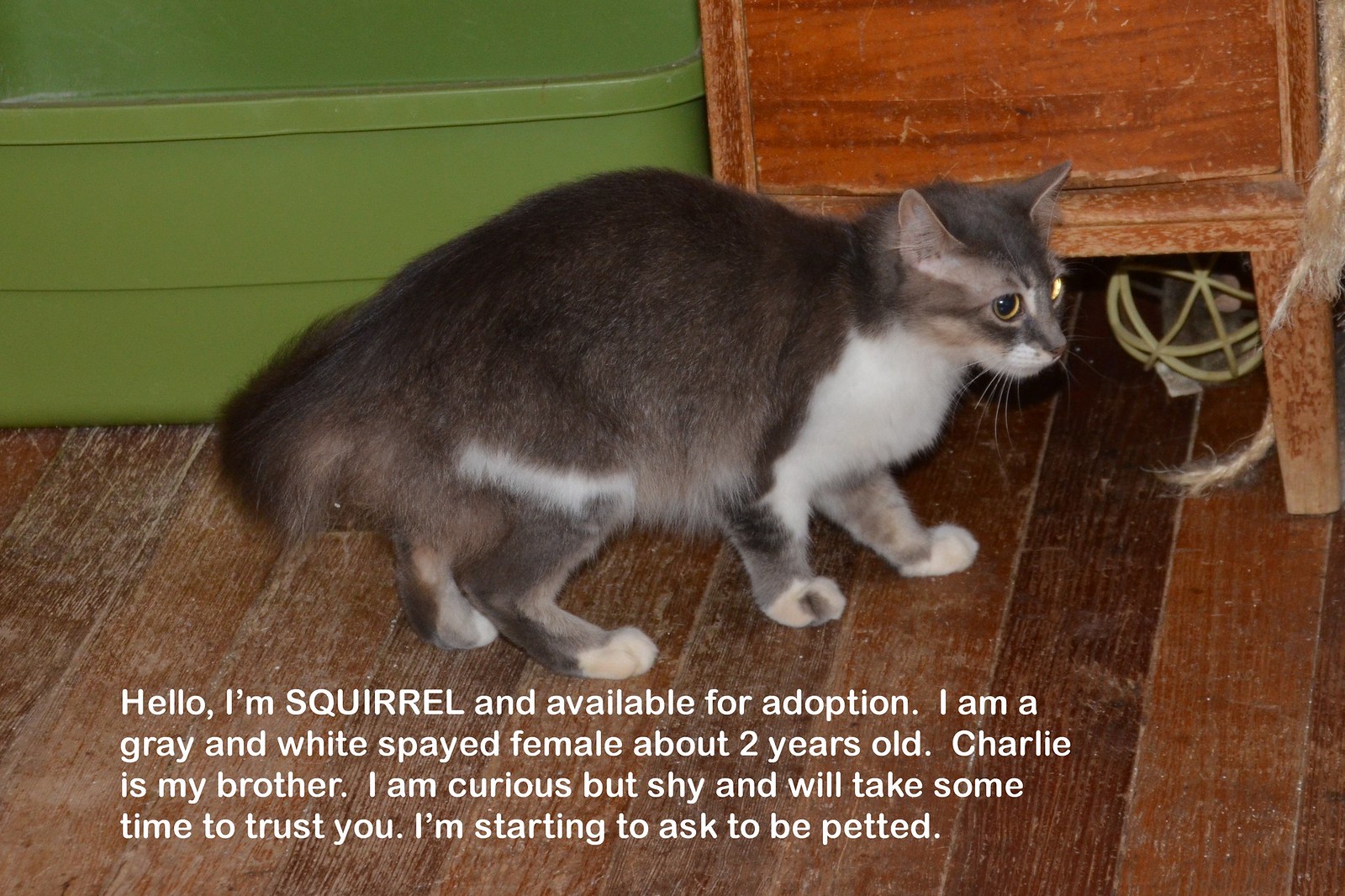In this photograph, a grayish-brown cat with a white underbelly, chest, whiskers, and paws stands on a worn wooden floor. Situated behind the cat on the right is a piece of aged wooden furniture, while a green plastic tub, possibly a cat box with sand, is visible on the left. The background also includes a white storage cabinet, with a cat toy peeking out from underneath. The bottom of the image features white text that reads: "Hello, I'm SQUIRREL and available for adoption. I am a gray and white spayed female, about two years old. Charlie is my brother. I am curious but shy and will take some time to trust you. I am starting to ask to be petted."